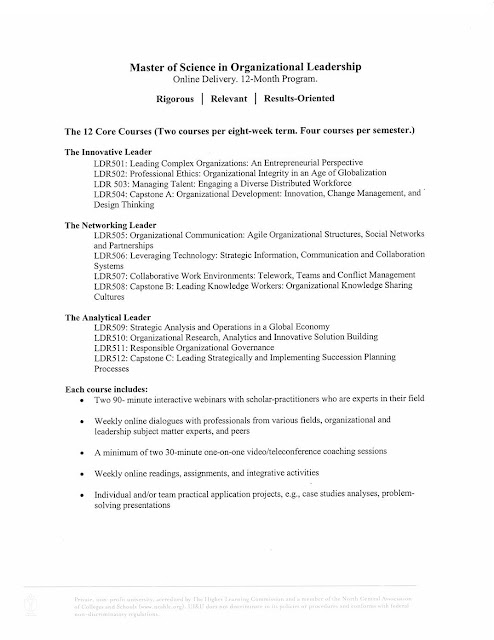This image outlines the pathway to earning a Master of Science in Organizational Leadership through a rigorous, relevant, and results-oriented 12-month online program. The entire page features black text on a white background. It details the 12 core courses, which are structured into two courses per eight-week term and four courses per semester. The program offers different tracks, namely the Innovative Leader, the Networking Leader, and the Analytical Leader, each comprising four specific courses designed to develop respective competencies. Example courses include LDR 501: Leading Complex Organizations and Entrepreneurial Perspective.

At the bottom, the page highlights key components of the program:

- Two 90-minute interactive webinars per course, featuring scholar practitioners who are experts in their field.
- Weekly online dialogues with professionals from various sectors, as well as organizational and leadership subject matter experts and peers.
- A minimum of two 30-minute one-on-one video teleconference coaching sessions throughout the program.
- Weekly online readings, assignments, and integrative activities.
- Individual and team practical application projects, such as case studies, analyses, and problem-solving presentations.

This structured and comprehensive program aims to equip students with the essential skills and knowledge necessary to excel in leadership roles.